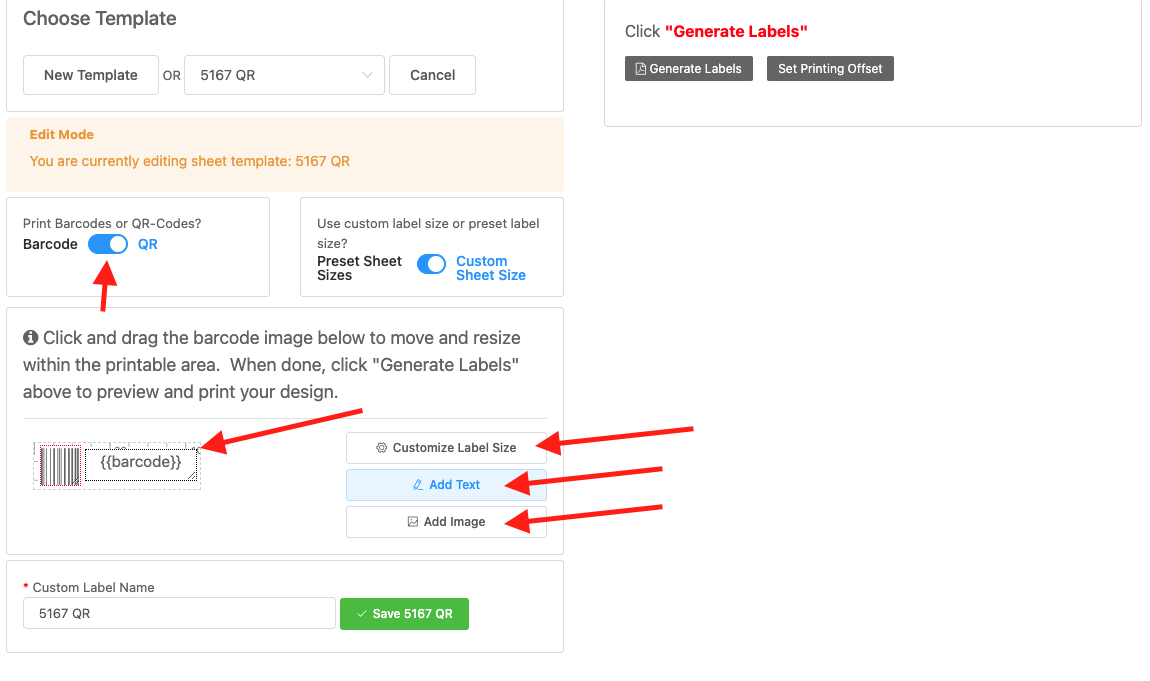Screenshot of a Website Tutorial Overview: 

The screenshot captures a webpage designed for a tutorial or guide, showcasing various functionalities of the site. The header reads "Choose Template," with adjacent entry fields. One field displays "New Template," while the other reads "5167 QR." Below, there's a "Cancel" button.

A highlighted segment with a tan background and orange text reads, "Edit Mode: You are currently editing sheet template 5167 QR." This section indicates that the user is working on a specific template.

Several red arrows are scattered across the page, pointing to key interactive elements, suggesting a walkthrough or instructional overlay. Noteworthy features include a blue toggle button labeled "Print Bar Codes or QR Codes," highlighted by an arrow pointing upward.

Adjacent to this, another segment offers options to "Use Custom Label Size" or "Preset Label Size," controlled by a blue toggle button, which is currently set to "Custom Sheet Size." Overall, the page appears to guide the user through customizing and managing template settings on the website.